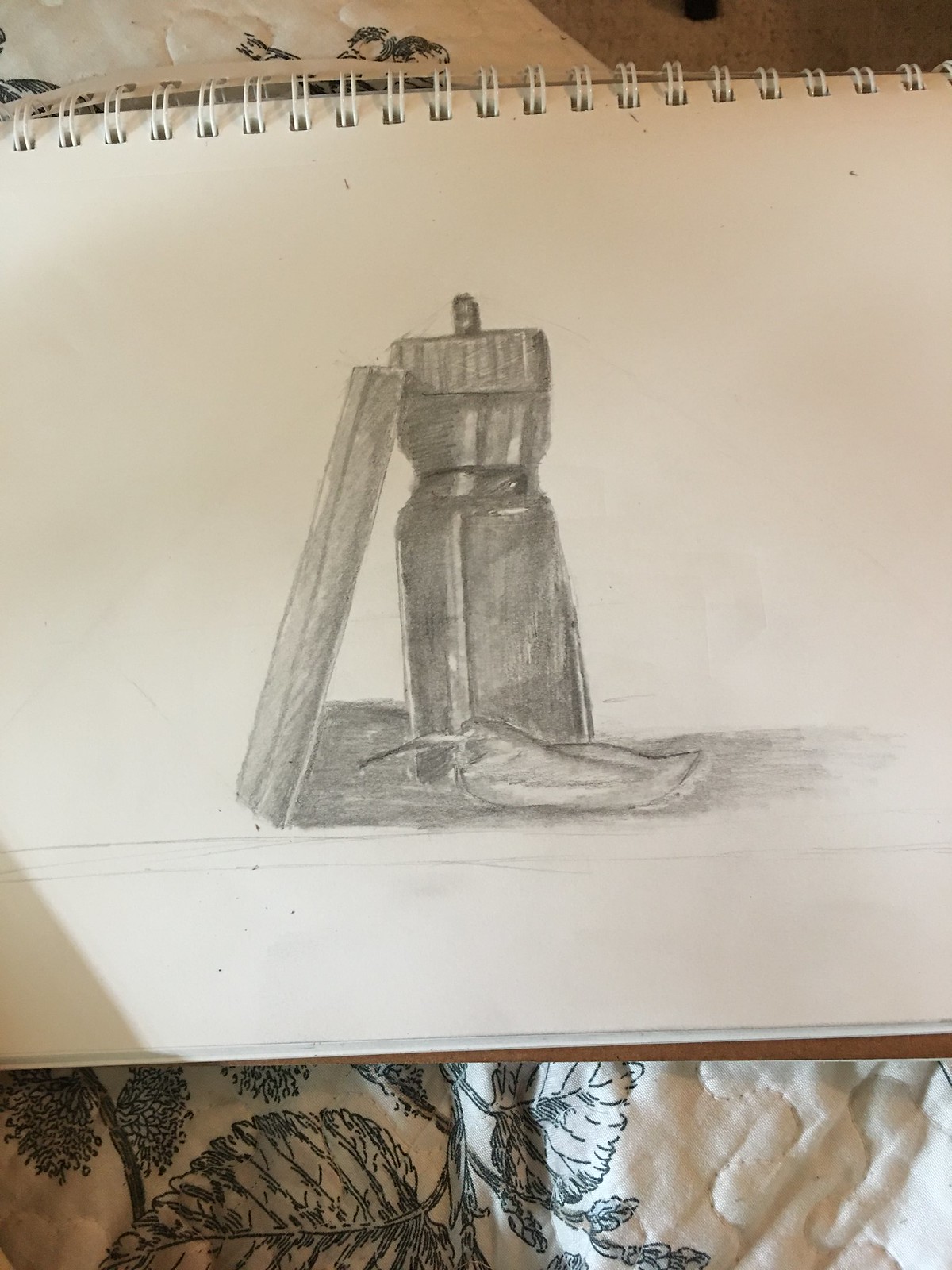A detailed sketchbook drawing depicts a cylindrical pepper grinder rendered meticulously with pencil. The shading varies, highlighting the grinder’s metallic texture and the object's contours. Leaning against the top of this pepper grinder is a rectangle-shaped object, enhancing the sense of depth. At the base of the grinder lies a small, slender pepper, likely a jalapeno, which is illustrated horizontally as a distinct, narrow rectangle. The image showcases a gradient of shading and intricate shadowing, bringing a realistic touch to the sketch.

The sketchbook itself has a noticeable spiral binding, possibly metal coated with white paint or encased in white rubber. The background of the photo reveals a white bedspread adorned with black plant motifs. Part of a carpet is visible, indicating the image was captured in a well-lit room, with a miscellaneous black object slightly left of the upper right corner, possibly a piece of furniture or another household item lying on the floor.